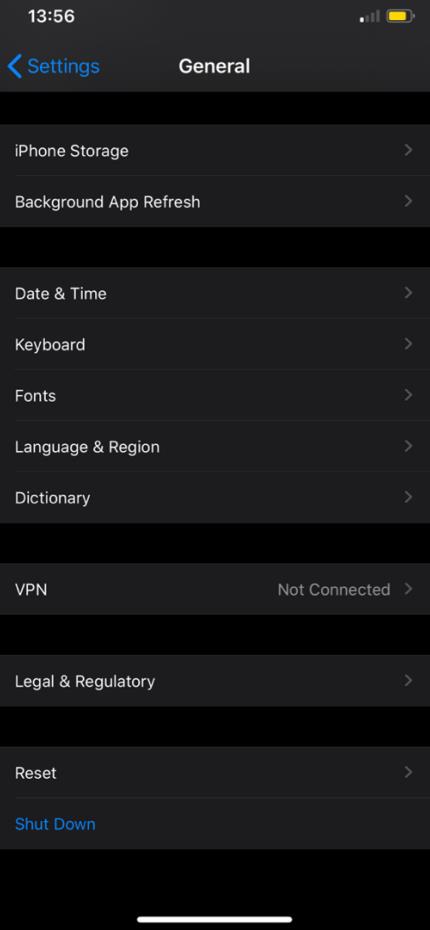This image depicts a settings page on a smartphone. The status bar at the top of the screen displays the time as 13:56 on the left, accompanied by a connection icon and a battery indicator on the right. The battery is approximately 80% charged, indicated by a yellow bar.

The interface features a dark gray background with alternating rectangular sections of varying shades, primarily dark gray and black. The top navigation bar showcases "Settings" in blue text on the left and "General" in white text in the center.

The main section of the page lists several categories aligned on the left-hand side, arranged from top to bottom as follows:

1. iPhone Storage
2. Background App Refresh
3. Date & Time
4. Keyboard
5. Fonts
6. Language & Region
7. Dictionary
8. VPN (not connected)
9. Legal & Regulatory
10. Reset
11. Shut Down (in blue text)

The very bottom of the screen has a black background with a single horizontal white bar in the center.